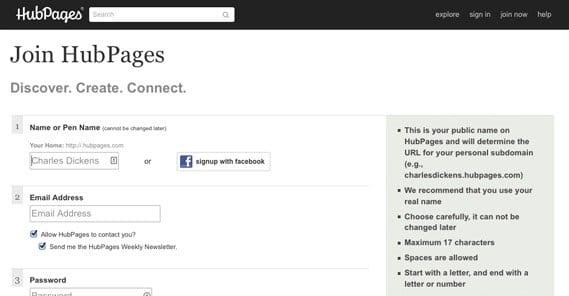The image features a predominantly black background with a sleek, user-friendly interface for the website "HubPages." On the left side, in elegant white cursive text, "HubPages" is written. Below that, a white rectangular search box displaying the word "Search" in gray allows users to look up specific content.

Towards the right of the image, four options are presented in gray lowercase letters: "explore," "sign in," "join now," and "help."

The main focus of the image appears to be a white page overlay, featuring black text. At the top left, the heading reads "Join HubPages" in black, with the tagline "Discover. Create. Connect." written in gray beneath it. Below this, there is a form asking for "Name or Pen Name," pre-filled with the example "Charles Dixon."

The form continues to request an email address, with checkboxes already ticked, granting permission for HubPages to contact the user and send weekly newsletters. There is also a field for entering a password, though this part of the image is cut off.

On the right-hand side, against a gray background with black text, the image explains that "Your public name on HubPages will determine the URL of your personal subdomain" (e.g., CharlesDixon.HubPages.com). The guidelines indicate that the name should be carefully chosen as it cannot be changed later. The name should be a maximum of 17 characters, can include spaces, and must start with a letter and end with a letter or number.

Overall, the image effectively showcases the HubPages sign-up process, emphasizing the importance of the user's chosen name and providing a clean, inviting interface.